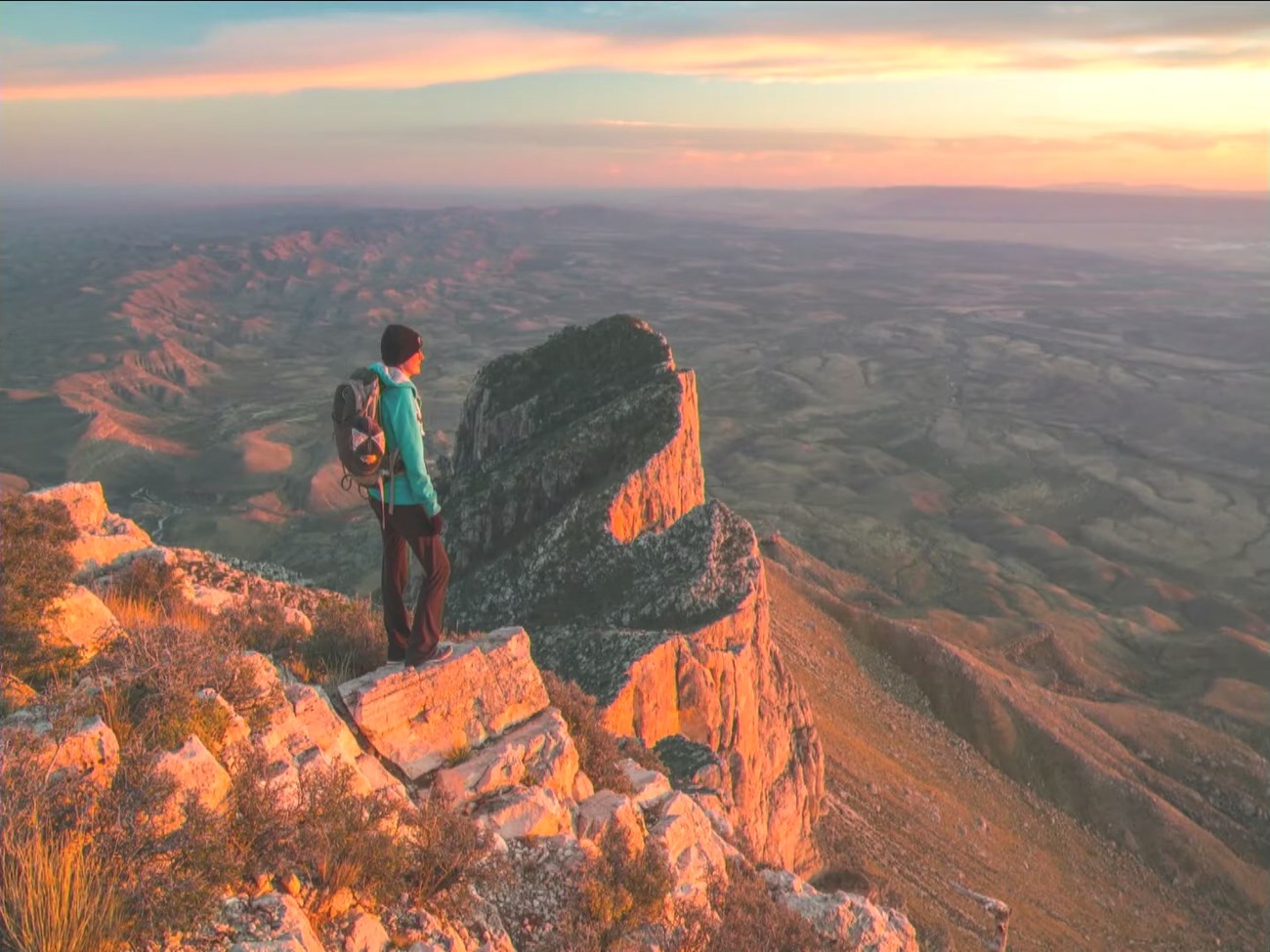The image is a stunning, professionally captured, outdoor color photograph taken from the summit of a mountain. At the forefront of the picture, towards the left, stands a hiker wearing a black hat, blue sweatshirt or jacket, black pants, and tennis or hiking shoes, along with a backpack. The hiker is standing on a stone outcropping, gazing over a vast, arid-looking canyon reminiscent of the Grand Canyon but not as deep. The sky above is a gorgeous tapestry of sunlight filtering through clouds, with hues of orange, yellow, and red suggesting the sun is either rising or setting. The photograph features muted natural tones, with the sun off to the right, highlighting the expansive view of the valley below and the distant backbone of a mountain range. The scene has a serene yet majestic quality, with the low-level plants and barren landscape adding to the rugged beauty of the canyon.